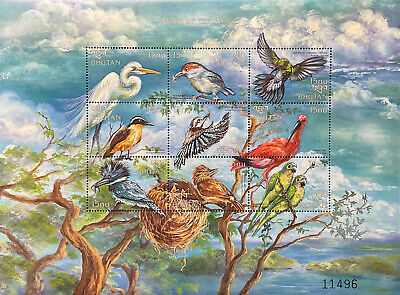The image portrays a vintage postcard-sized sheet of postage stamps from Bhutan, featuring a collage of nine rectangular stamps with perforation lines. Each stamp illustrates a different exotic bird perched on or flying around a green leafy tree with a brown trunk. The birds are mainly white, blue, yellow, orange, and green in color. In the background, a painted sky filled with white and blue clouds complements a seascape in the bottom right corner. The detailed scene also includes a nest positioned centrally in the tree. The stamps collectively form a cohesive illustration of this natural scene, rather than just individual images. The text "Bhutan" is visible on each stamp, and the sheet bears the serial number 11496 in the lower right corner.